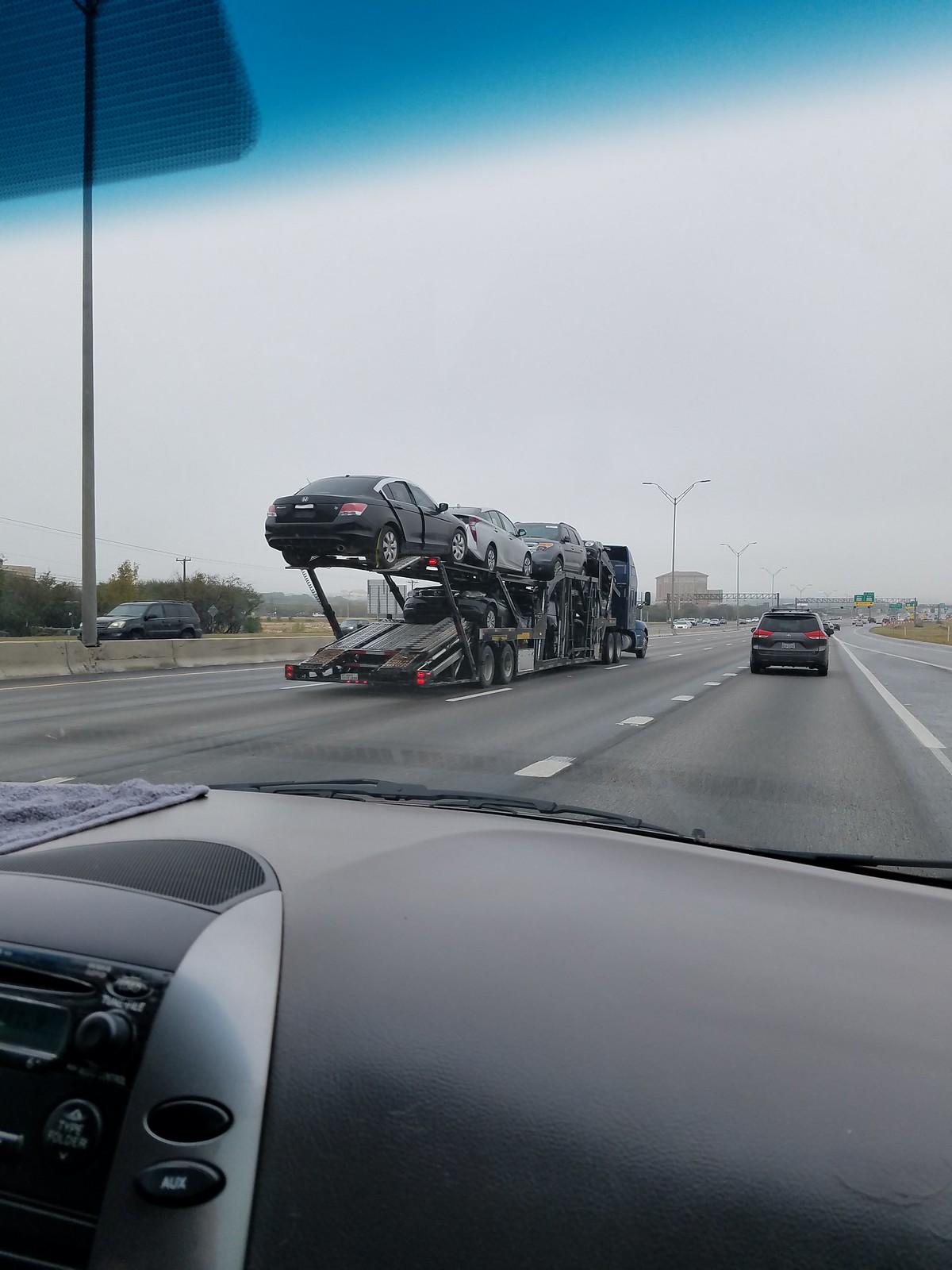The photograph captures the view from inside a vehicle traveling on a four-lane highway on an overcast day. Taken from the passenger seat, the dashboard and part of the car's center control panel are visible, including the tinted top portion of the windshield. The freeway is relatively empty, with well-spaced, smoothly flowing traffic. In the foreground, a black vehicle directly ahead is followed by an SUV further up with red taillights. Two lanes over, a trailer truck is transporting five to six cars, some stacked on the lower level while the upper level is fully loaded with a mix of black, white, and silver cars. The scenery outside features some low buildings, gray lamp posts, and green and yellow traffic signs. The sky is heavily clouded, contributing to the overall grayish tone of the photograph. The pavement details, including white dotted lane markings, are clearly visible, and there's a concrete divider separating the lanes with occasional glimpses of traffic moving in the other direction. No significant landmarks stand out in the distance, providing a typical freeway setting.